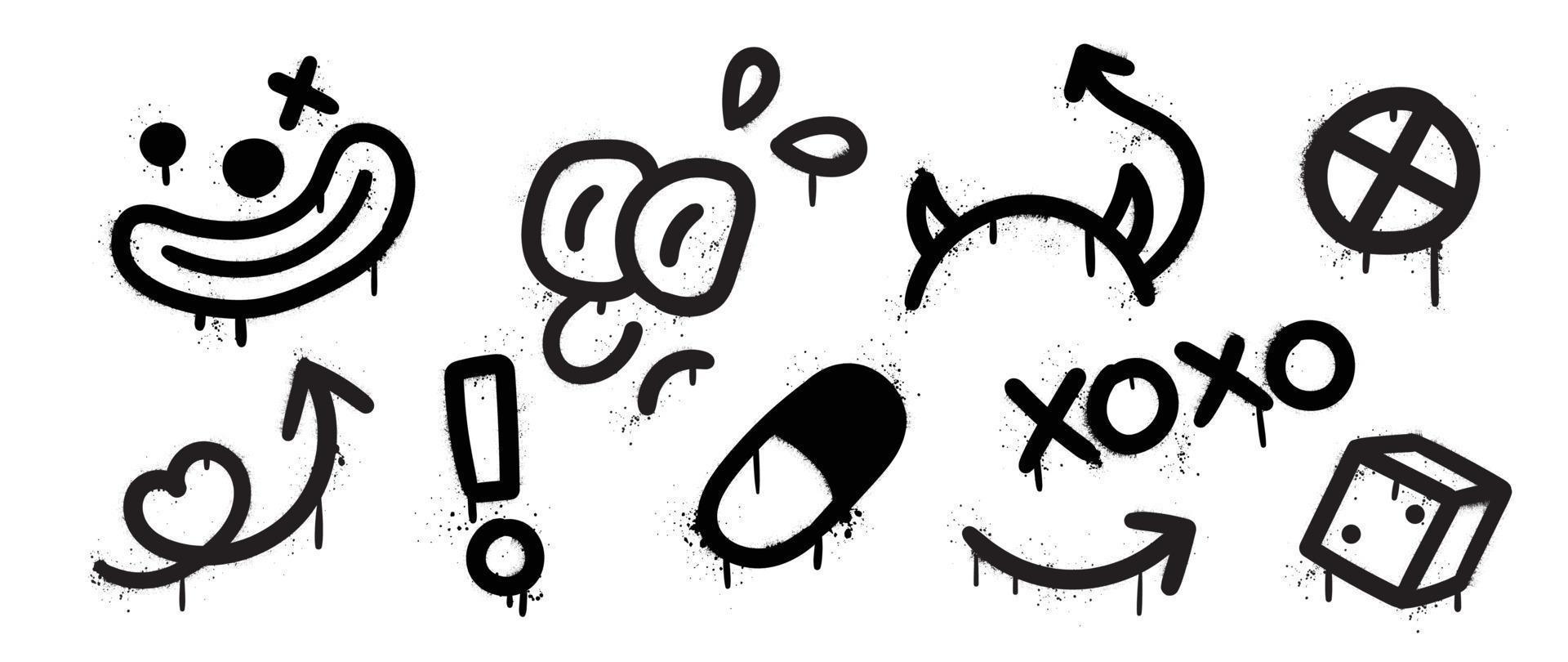This image features a collection of highly detailed black and white spray-painted doodles and cartoons on a white background. At the top, there are four distinct illustrations from left to right: a clownish face comprising two eyes (one marked with an X) and a wide mouth; a face with bulging eyes and what seem to be eyebrows or splashes of water, giving it an anxious look; a rounded head with possible devil-like or cat ears, and a tail ending in an arrow tip; and finally, a circle intersected by an X. 

The bottom row showcases five more drawings: a heart pierced by an arrow in a continuous line; a stylized exclamation point; a pill split into black and white halves; XOXO with an arrow pointing right below it; and a cube that could be interpreted as either a die showing the number two or a sugar cube. The entire composition of doodles appears as if they were spray-painted, complete with drips and spray marks to accentuate the graffiti style. The image lacks any signatures or text.